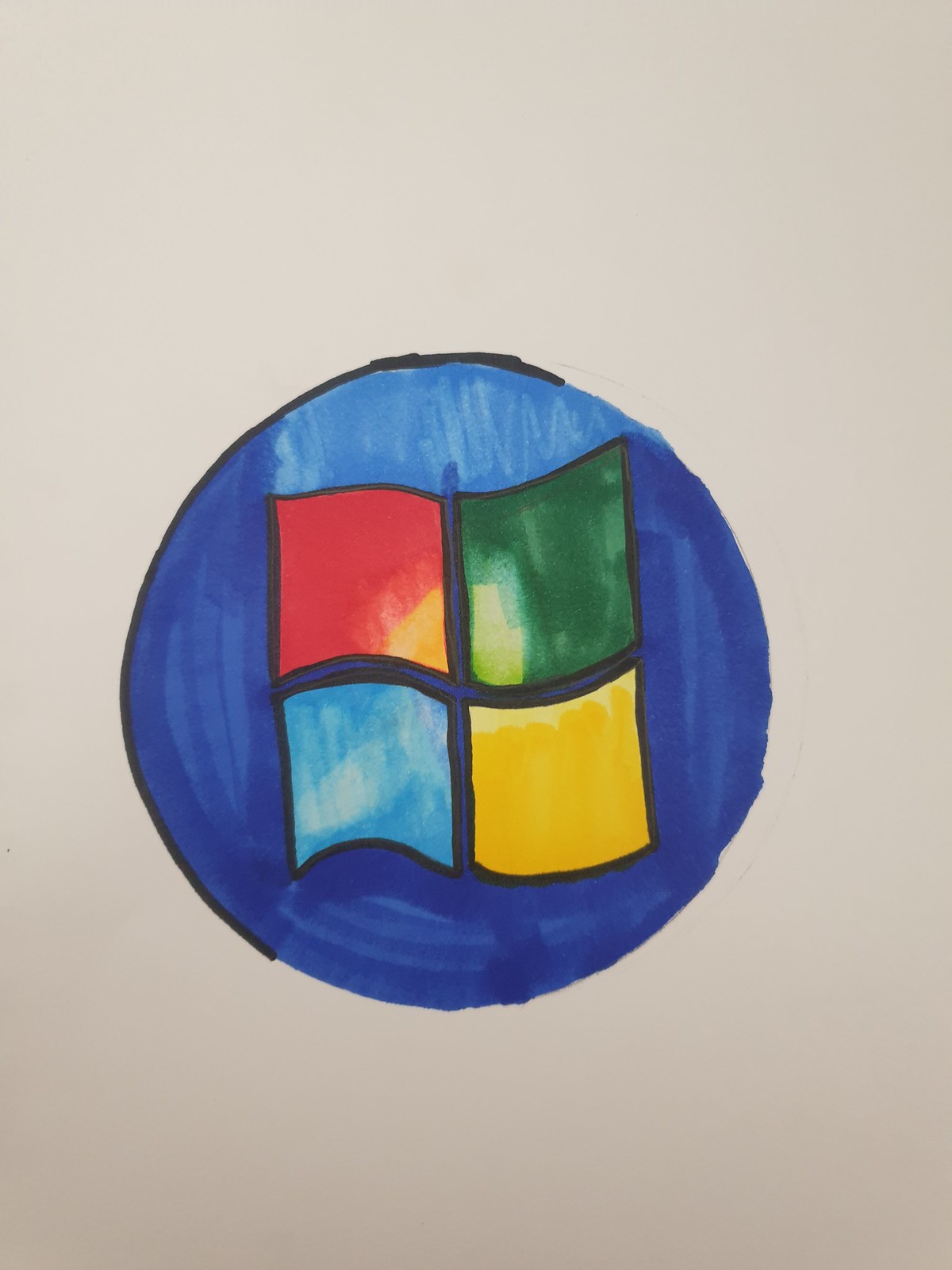The image features a gray background with a dark blue circle at the center, framed by a black border. Prominently displayed within the circle is the Windows symbol, comprised of four wavy squares. The top left square is red, the top right square is green, the bottom left square is light blue, and the bottom right square is yellow. Notably, the top left square and bottom right square have a uniform color intensity, whereas the top right and bottom left squares appear lighter, giving the effect of being drawn with a marker.